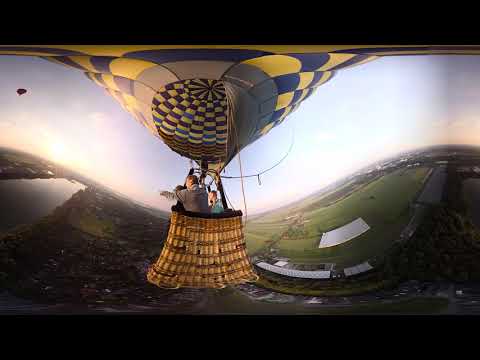The image captures a hot air balloon flight with a nearly centered wicker basket. The basket is woven in shades of brown and light beige, with the intricate weaving clearly visible. Inside the basket, there are three figures facing away from the camera. The primary figure on the left wears a long-sleeved gray shirt and points toward the left. Partially obscured by this figure, another person dressed in dark clothing is visible. To the right, a third figure with long blonde hair wears a light aqua jacket. Above them, the hot air balloon's blue and yellow checked pattern is evident.

The scene below unfolds into a panoramic view, revealing expansive fields, a long grassy area, and a rectangular body of water that resembles a man-made lake. On the far left, a river and more green terrain can be seen. There’s also a long building with a white roof, possibly part of a farm which includes a stable-like structure. The day is partly cloudy with occasional breaks of sunshine. In the upper left distance, another hot air balloon floats in the sky. The entire image is framed with a thick black border at the top and bottom.